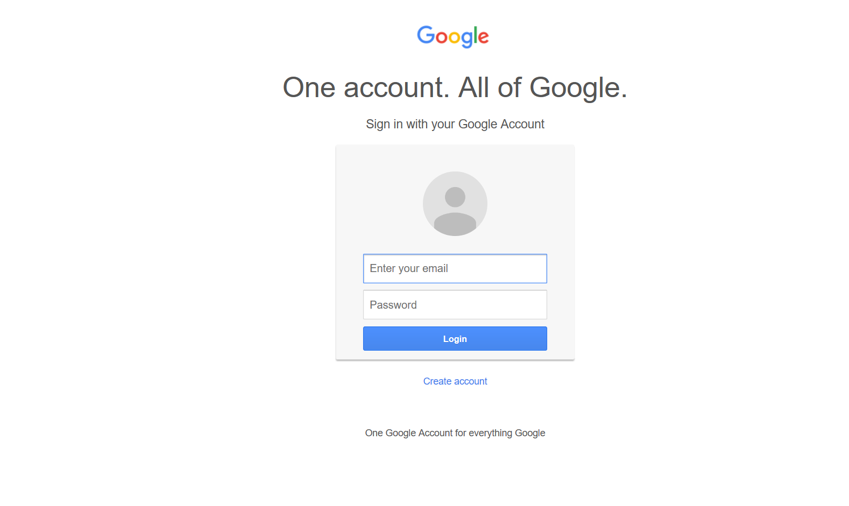Screenshot of the central section of a webpage. The background is entirely white, with no discernible boundaries. At the top, the Google logo is prominently displayed, featuring the iconic multicolored letters: a blue "G," a red "o," a yellow "o," a blue "g," a green "l," and a red "e." Below the logo, the text reads in black, "One account. All of Google." Following this, a smaller black font instructs users to "Sign in with your Google Account."

Beneath the text, there is a small gray box displaying a people icon, which comprises a dot atop an oval within a circle. Below this, two text input fields are present. The top field, highlighted in blue, prompts the user to "Enter your email," while the bottom field is labeled "Password." Adjacent to these fields, a rectangular "Log in" button is shown with a blue background.

Near the bottom of the screenshot, the options "Create account" in blue text and further below, in black, the phrase "One Google Account for everything Google."